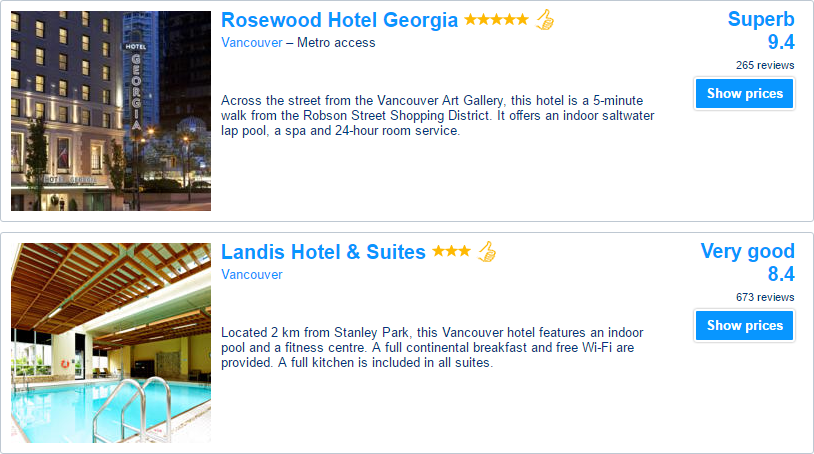The image features a dual screenshot from a travel website, highlighting two different hotels. The upper section of the image focuses on the luxurious Rosewood Hotel Georgia, with visuals depicting the building illuminated at night. 

**Left Side:** 
- An image of Hotel Georgia at night.
- A descriptive paragraph reads: "Across the street from the Vancouver Art Gallery, the hotel is a five-minute walk from the Robson Street Shopping District. It offers an indoor saltwater lap pool, a spa, and 24-hour room service."

**Right Side:**
- "Rosewood Hotel Georgia" is prominently displayed with five stars beneath it.
- Location: Vancouver, with the additional note "Metro access."
- Guest Rating: "Superb" with a score of 9.4 based on 265 reviews.
- A blue rectangle button labeled "Show prices."

The lower section of the image spotlights the Landis Hotel and Suites, focusing on an inviting pool area, with visible steps leading into the water.

**Left Side:**
- A picture highlighting the distinctive pool of the Landis Hotel and Suites.

**Right Side:**
- "Landis Hotel and Suites" labeled with three stars and a thumbs-up icon.
- Location: Vancouver.
- Guest Rating: "Very good" with a score of 8.4 based on 603 reviews.
- A blue rectangle button labeled "Show prices."
- A descriptive paragraph follows but is not fully visible in the screenshot.